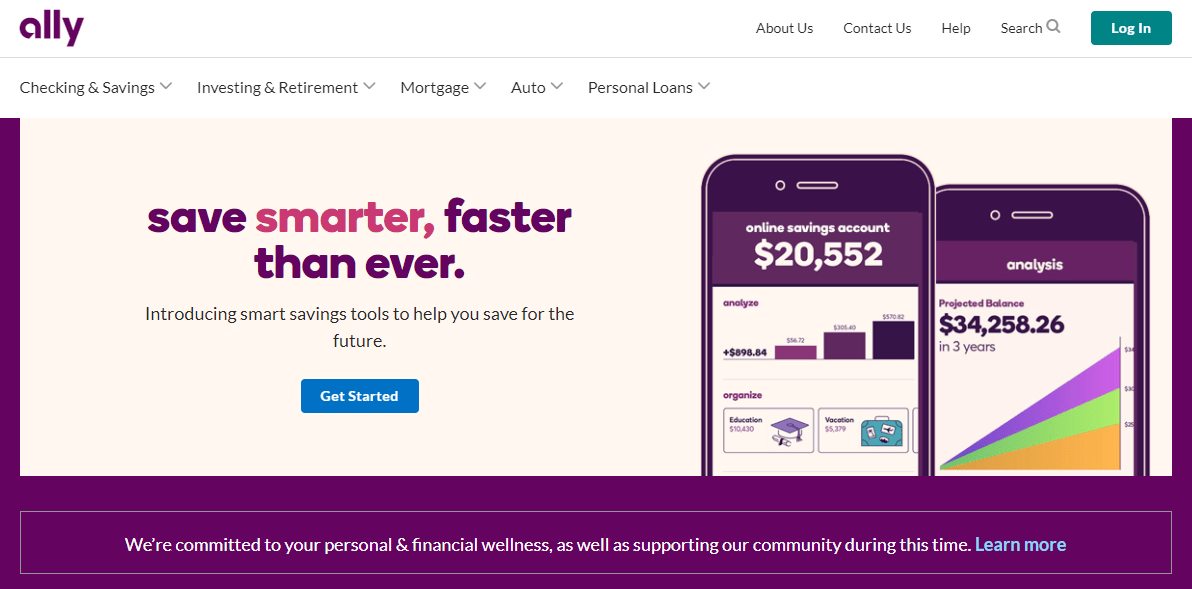The image is a horizontally rectangular screenshot from the Alley Bank website. In the upper left corner, the purple Alley company name is prominently displayed. On the right side, against a white background, black text links read About Us, Contact Us, Help, and Search, positioned beside a green Login button. Below the company name "Alley" on the left, there are several drop-down menus labeled Checking and Savings, Investing and Retirement, Mortgage, Auto, and Personal Loans. 

Beneath these menus, there is an eye-catching advertisement that states, "Save Smarter, Faster Than Ever. Introducing Smart Savings Tools to Help You Save for the Future." Centrally located below this message is a blue, horizontally rectangular button with the text "Get Started" in white.

On the right side of the image, two partially visible cell phones display representative windows from Alley's mobile application. The left cell phone shows "Online Savings Account: $20,552" with some analysis data below it. The right cell phone displays "Analysis: Projected Balance: $34,258.26 in three years," providing an overview of the account's future projections.